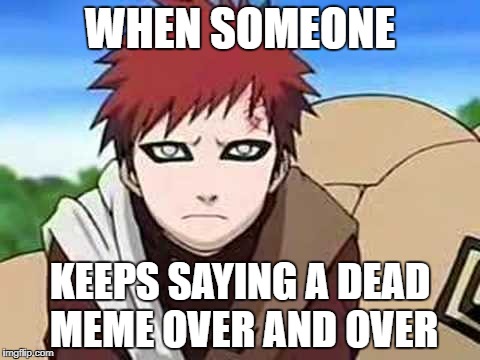The image is a detailed color illustration in a manga anime style, presented in landscape orientation. The central character is a young male with striking red spiky hair and intensely outlined black eyes, exuding an upset, disappointed expression as he leans forward and glares at the viewer. His mouth is set in a frown, encapsulating his frustration. He is adorned with a beige patch over his left shoulder and a cream-colored scarf draped over his right. Behind him, to the right, there is a mound-shaped beige object. The background features a serene blue sky and green trees, situating the scene outdoors. The image contains white text overlayed at the top and bottom, reading, "When Someone Keeps Saying a Dead Meme Over and Over." In the bottom right corner, the credit "imageflip.com" is visible.